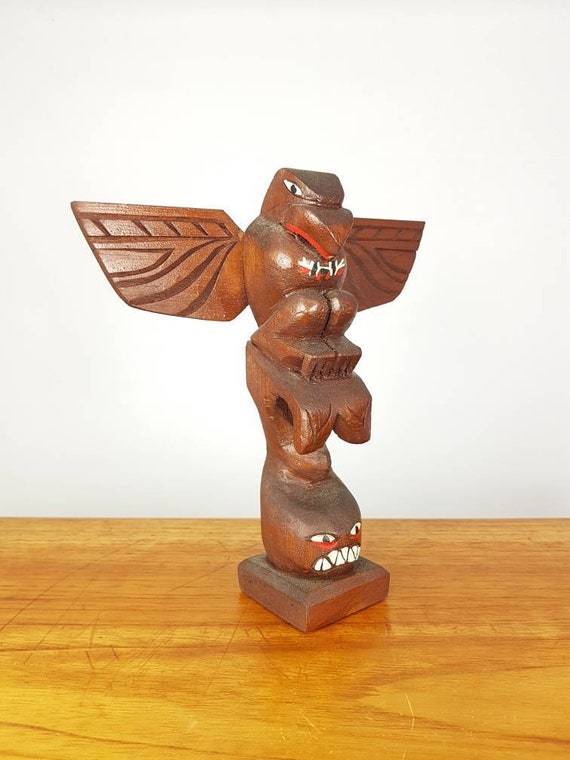The image features a small, intricately carved wooden totem pole made of dark walnut-colored wood, positioned on a light brown wood tabletop, which has visible scratches and a distinct wood grain pattern. The totem pole includes two main figures: a bird, possibly an eagle, perched at the top with outstretched wings, and a creature resembling a whale at the base. The whale is depicted with a face showing sharp teeth and two eyes, giving it a glaring expression. Its tail is bent forward beneath the bird, forming part of the structure that supports the avian figure above. The bird has a stern look in its eyes, a beak painted slightly orange, and a unique design on its chest featuring red, white, and black patterns that evoke a Native American or possibly Polynesian style. The entire sculpture is well-lit against a white wall, and its small size suggests it could fit in one's hand.